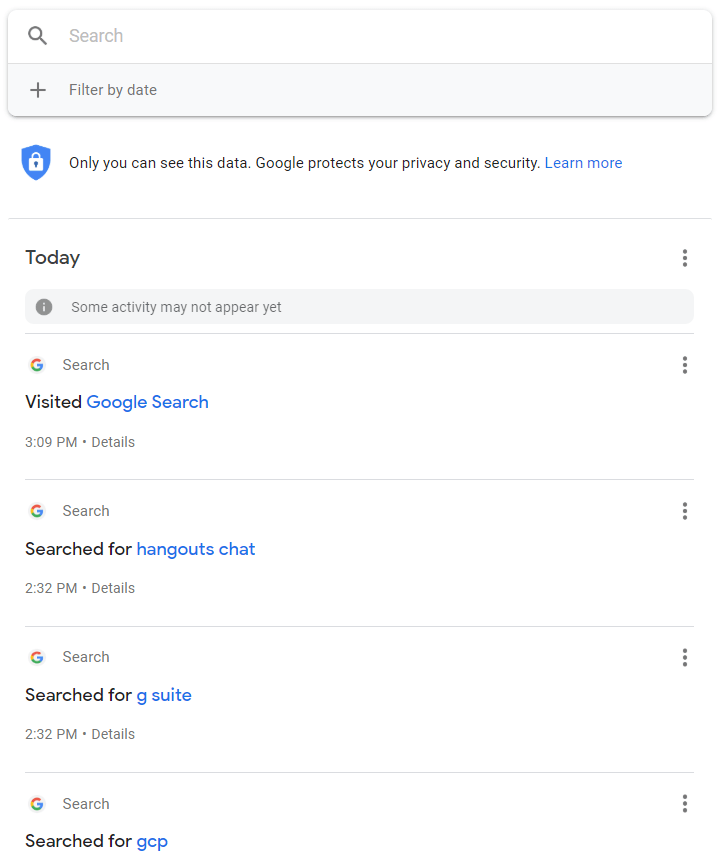The illustrated image depicts a user's Google search history page. At the top of the page is a search box featuring a magnifying glass icon. Below it, there is a "Filter by date" option accompanied by a plus sign.

Directly underneath, there is a blue shield icon with a white lock inside it, next to a message reassuring the user: "Only you can see this data. Google protects your privacy and security." Additionally, the phrase "Learn more" appears in blue, indicating it is a clickable link.

Moving further down, a "Today" section is highlighted, which includes three vertical dots on the right side, signifying additional options. Beneath this section, a note states, "Some activity may not appear."

Following this, individual search entries are listed. The first entry shows a search conducted at 3:09 PM with the label "Visited Google search," and an associated "Details" link. The subsequent entries sequentially list other searches: "Search for hangouts chat" at 2:32 PM, "Search for G Suite" at 2:32 PM, and "Search for GCP" with each entry including corresponding times, "Details" links, and three vertical dots for each, suggesting further actions or information.

The interface is primarily white with black text, while key elements and links, such as "Learn more" and specific search times, are highlighted in blue for emphasis. The Google logo is present next to the search entries, reinforcing the source of the searches. Overall, the clean and straightforward layout indicates that the user is browsing their Google search history, likely in pursuit of particular information.